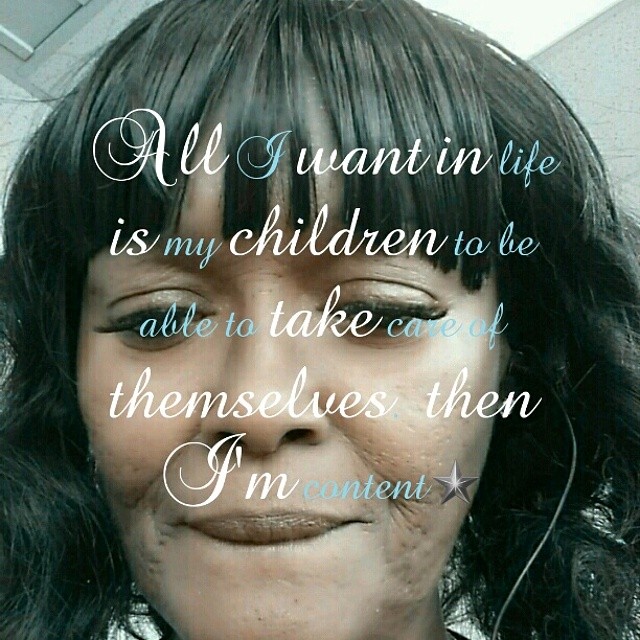The image is a color close-up photograph of an African-American woman with long brown, wavy hair. Her eyes are seemingly open but partially covered by overlaid text, making it hard to see clearly. Her upper lip is pressing down on her lower lip, and there's a black wire, likely from earplugs, visible coming out of her left ear. The background is a blend of gray and white. Superimposed over the image is a motivational quote in a white and blue cursive font, spanning five lines: "All I want in life is my children to be able to take care of themselves then I'm content." A small silver star follows the text. The overall tone of the photograph is intimate, capturing the woman's reflective expression.